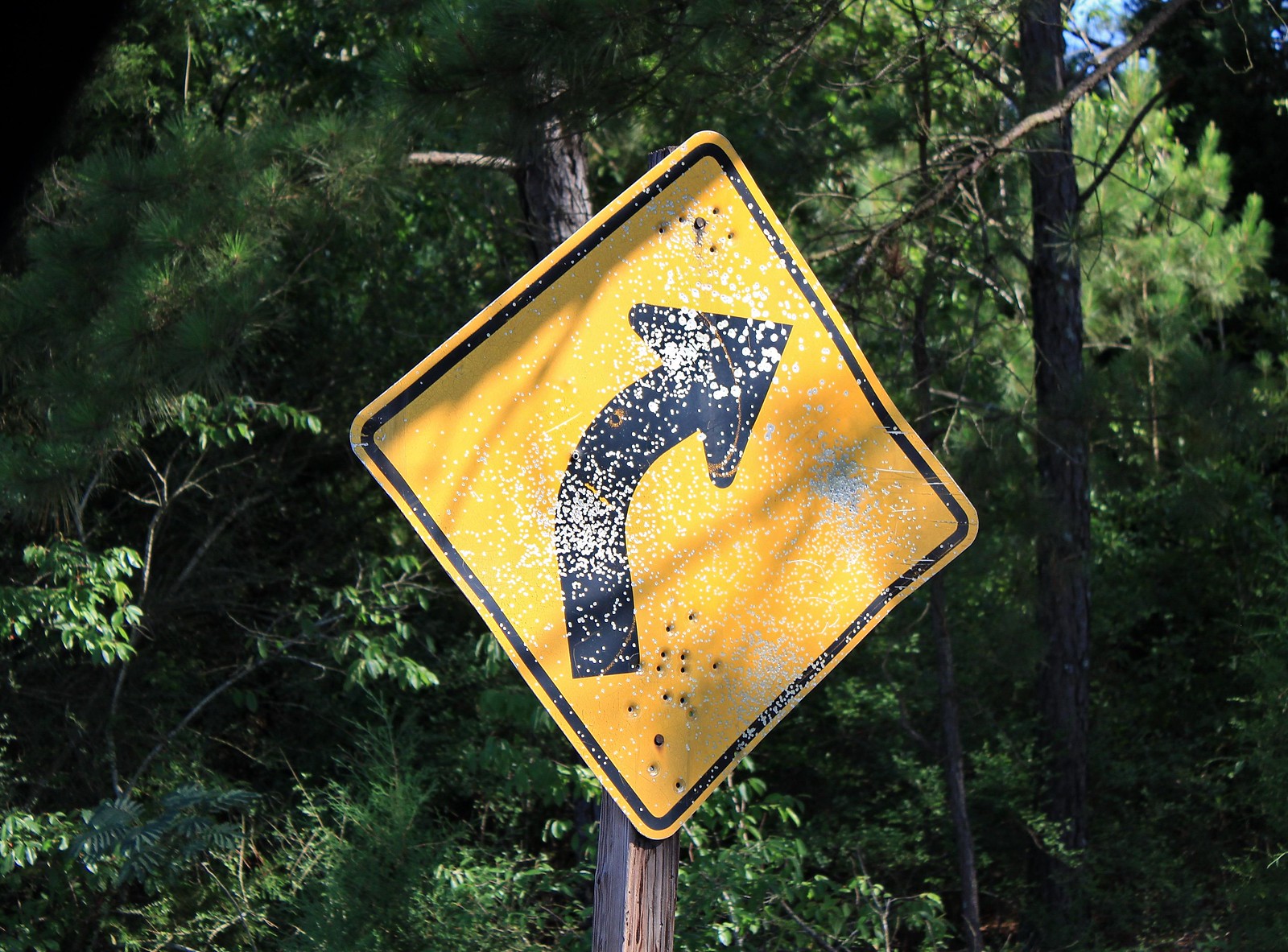The daytime outdoor color photograph captures a yellow diamond-shaped street sign with a black border and an upward-pointing black arrow angled to the upper right, indicating an upcoming right curve. This well-worn metal sign, marred by missing paint specks and what appear to be BB gun holes, is mounted on a wooden post that extends out of the bottom of the image. The right tip of the sign is slightly bent. The surroundings include a dense forest featuring a mix of tree trunks, bright green leaves, and likely some pine trees, suggesting a summer setting. Sunlight from the upper right brightly illuminates the sign as well as parts of the vibrant foliage. A patch of blue sky is visible at the top-right corner, enhancing the image's natural beauty.